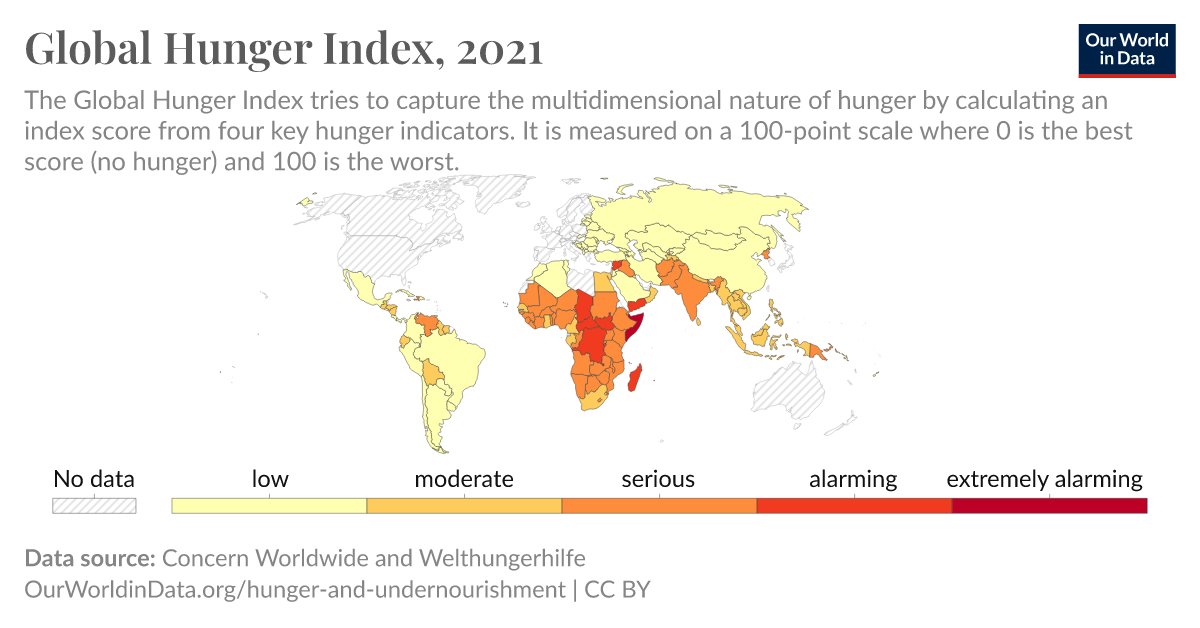The image depicts an educational infographic titled "Global Hunger Index 2021," presented by Our World in Data, Concern Worldwide, and Welthungerhilfe. The infographic is designed to illustrate the multidimensional aspects of hunger using a color-coded world map and is accompanied by a detailed explanation. The Global Hunger Index (GHI) scores countries on a 100-point scale, where zero represents no hunger and 100 indicates the highest level of hunger. 

The map uses a range of colors to indicate the severity of hunger: yellow represents low hunger levels, light orange for moderate, dark orange for serious, red for alarming, and burgundy for extremely alarming. Areas with no available data are shown with gray diagonal stripes. The map shows that the countries with the most alarming levels of hunger are predominantly located in Africa and the Middle East, while India, Pakistan, and some neighboring countries are marked as serious. Most of Europe, North America, Australia, New Zealand, Russia, China, Mongolia, and parts of South America are indicated as low. 

Additionally, a graph at the bottom categorizes countries based on their hunger severity. The data source is credited to Concern Worldwide, Welthungerhilfe, and ourworldindata.org.